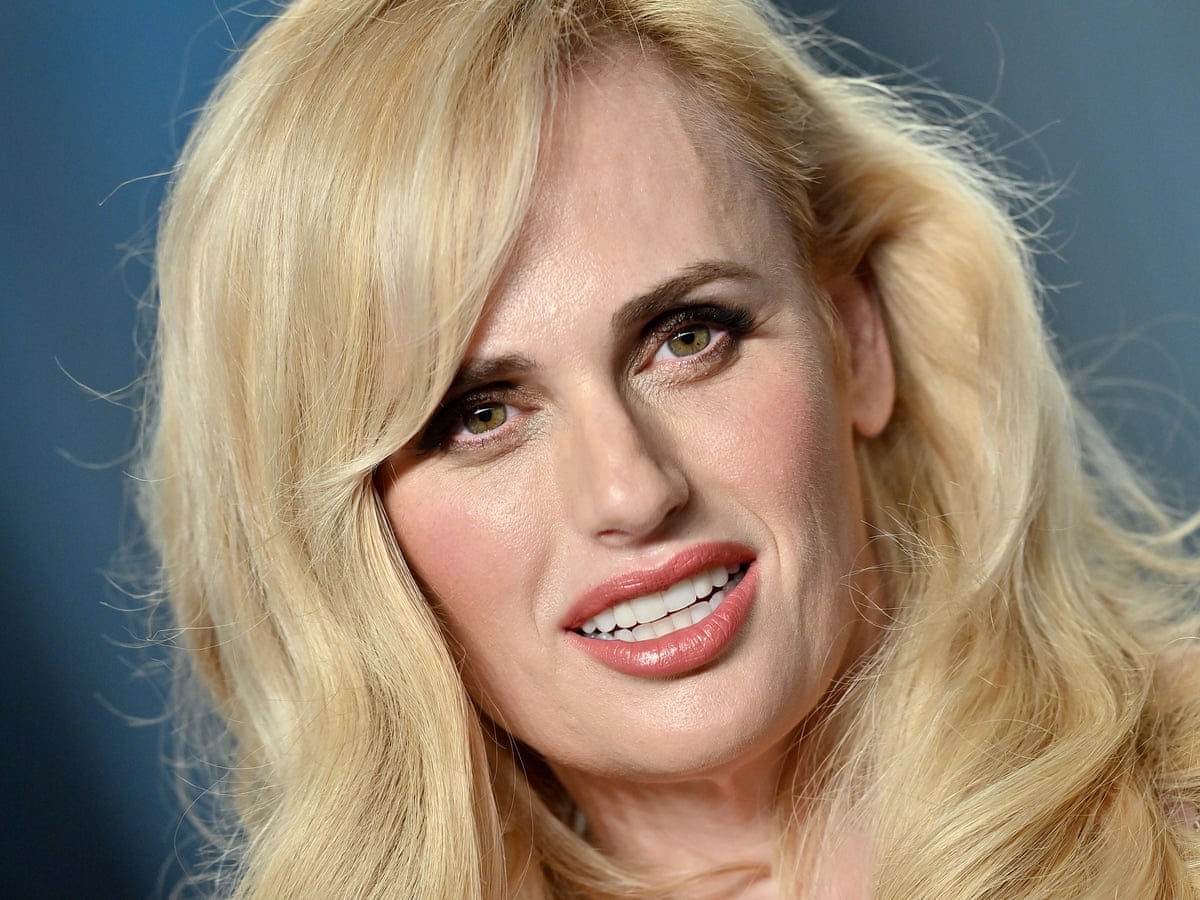The image showcases a close-up photograph of a young, blonde woman with long hair, possibly an actress or celebrity. Her hair, which reaches past her shoulders and features darker blonde accents, predominantly flows down her left side, while the right side is tucked behind her ear, revealing her left ear. She possesses striking green, hazel-like eyes that, in an almost Mona Lisa-esque manner, appear to be looking directly at you but are actually gazing slightly to the right. Her face is adorned with well-applied makeup, including dark eyebrows, a fair complexion, and peachy lipstick accompanied by matching blush on her cheeks. She is smiling, displaying her very white teeth, with her head slightly tilted to the right, enhancing the illusion. The background of the image is a blurred blue, providing a subtle contrast to her radiant skin and peach-pink lips. Additionally, there are faint wrinkles near her mouth, adding a touch of realism to her otherwise perfect appearance. The photograph captures her face prominently, extending from her neck up with just a hint of her right shoulder visible.